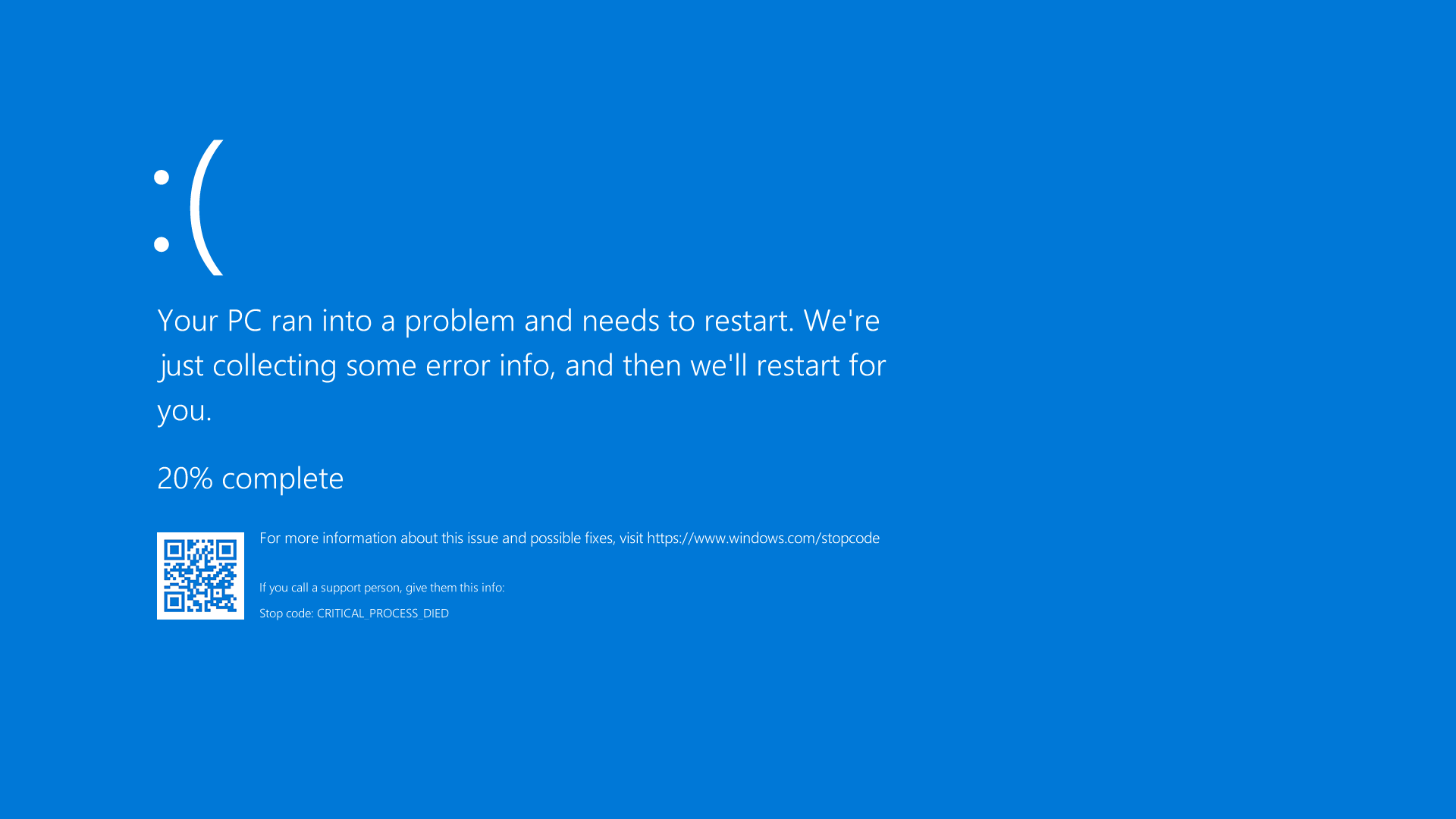The image is a Windows error message displayed on a PC, showing a blue background with white text. In the top left corner, there is a sad face emoticon, constructed using a colon and a parenthesis turned 90 degrees counterclockwise (resembling an upside-down smiley face). Below the sad face, the main text reads: "Your PC ran into a problem and needs to restart. We're just collecting some error info, and then we'll restart for you." Beneath this message, it indicates that the process is "20% complete." Directly under the percentage text, there is a QR code. Adjacent to the QR code, smaller text provides additional information: "For more information about this issue and possible fixes, visit https://www.windows.com/stopcode." Additional, barely readable text includes a stopcode labeled "CRITICAL_PROCESS_DIED", and there is some more text that is too small to discern. This image is commonly known as the Windows Blue Screen of Death, which appears when a critical error occurs in the system.